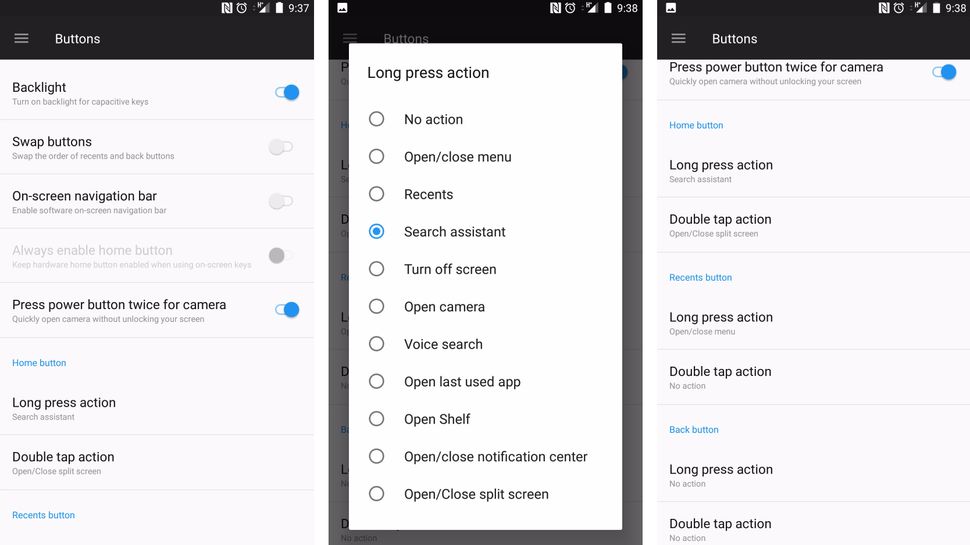This image consists of three screenshots of a mobile device's settings menu. 

**Left Screenshot:**
- **Top Bar:** A consistent black bar with a hamburger menu on the left, followed by icons for additional options, Chrome browser timestamp showing 9:37, 9:38, and 9:38 respectively, battery level indicator, and signal strength indicator.
- **Content:** The screen is titled "Admin Panel." The settings shown include:
  - **Backlight:** Enabled
  - **Swap Buttons:** Disabled
  - **On-Screen Navigation:** Disabled
  - **Always Enable Home Button:** Option is grayed out and disabled
  - **Press Power Button Twice for Camera:** Enabled
  - **Home Button:** Displayed in blue text
  - **Long Press Action & Double Tap Action:** Options are visible but not detailed here
  - **Recent Buttons:** Present but not specified further

**Center Screenshot:**
- **Pop-up Display:** A pop-up window titled "Long Press Action" with approximately 10-12 selectable options. Each option has a radio button on the left side. Options include:
  - No Action
  - Open/Close Menu
  - Recent
  - Search Assist (selected with a blue highlighted circle)
  - Turn Off Screen
  - Open Camera
  - Voice Search
  - Open Last Used App
  - Open Shelf
  - Open/Close Notification Center
  - Open/Close Split Screen

**Right Screenshot:**
- **Settings Display:** Similar to the left screenshot focusing on customization of action buttons:
  - **Press Power Button Twice for Camera:** Visible
  - **Home Button:** Displayed with options for Long Press and Double-Tap Actions
  - **Recent Button:** Options for Long Press and Double-Tap Actions
  - **Back Button:** Options for Long Press and Double-Tap Actions
  - The actions for the last three buttons (Home, Recent, and Back) at the bottom show "No Action" with some options for opening and closing menus or the Search Assistant.

Overall, the image provides a comprehensive view of the customization options available in the admin panel of the device's settings, focusing on button functionalities and specific actions for long press and double-tap commands.